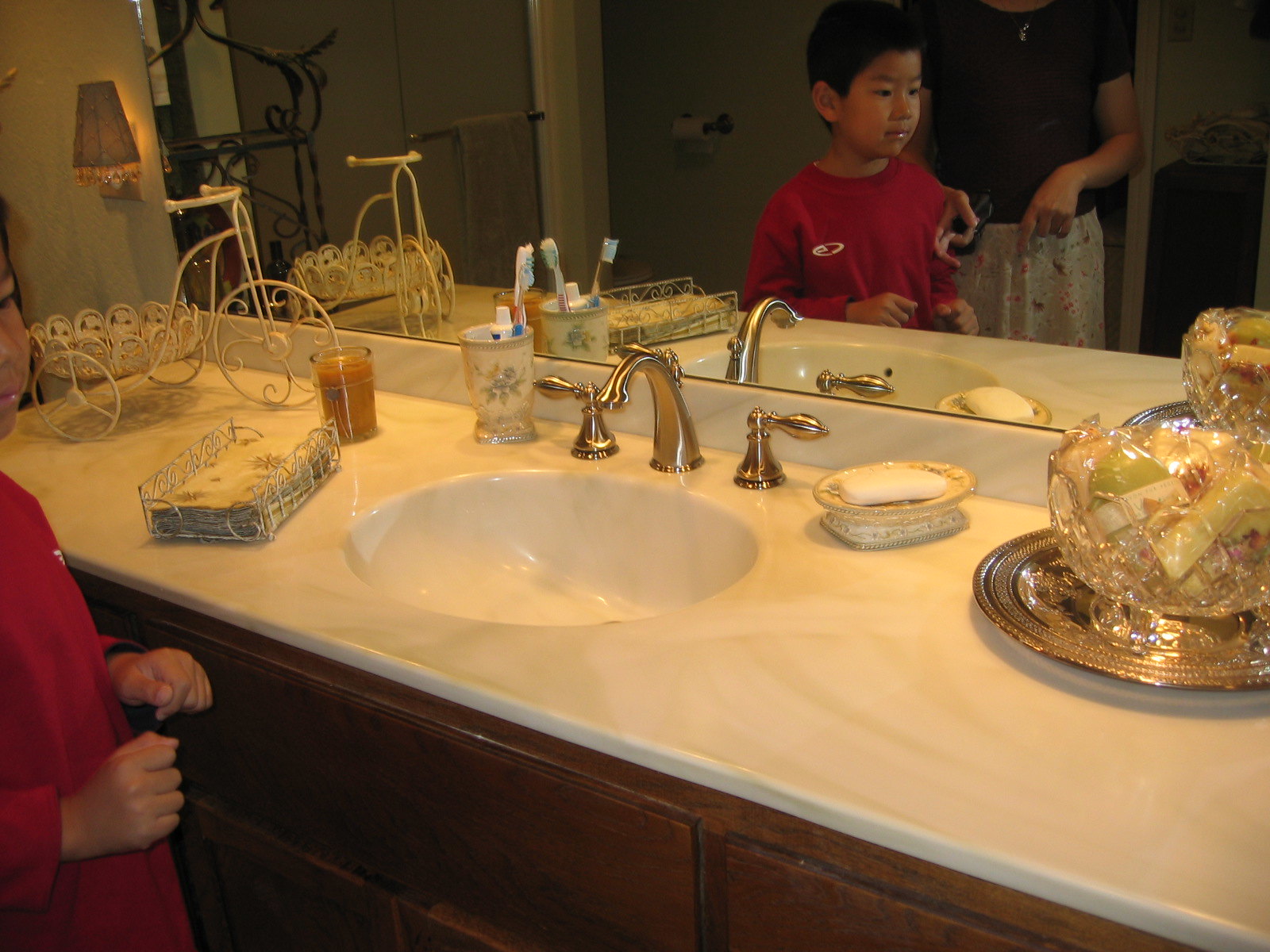The photograph captures an intricately decorated bathroom area. On the left side of the image, a child with dark hair, wearing a red shirt adorned with a white logo, is visible. His face is reflected in the mirror on the right side of the photo, revealing his East Asian features. Standing behind him, also visible in the mirror, is a woman dressed in a white skirt paired with a dark top and accessorized with a striking gold necklace. They are positioned in front of a spacious bathroom sink equipped with elegant gold faucets and water handles. Beside the sink, a gold tray holds a glass bowl filled with an array of soaps and hygiene products. A toothbrush holder containing toothpaste is also present, along with a metal basket stacked with neatly folded towels. The opulence of the bathroom decor is highlighted by the use of luxurious materials and thoughtful arrangements.